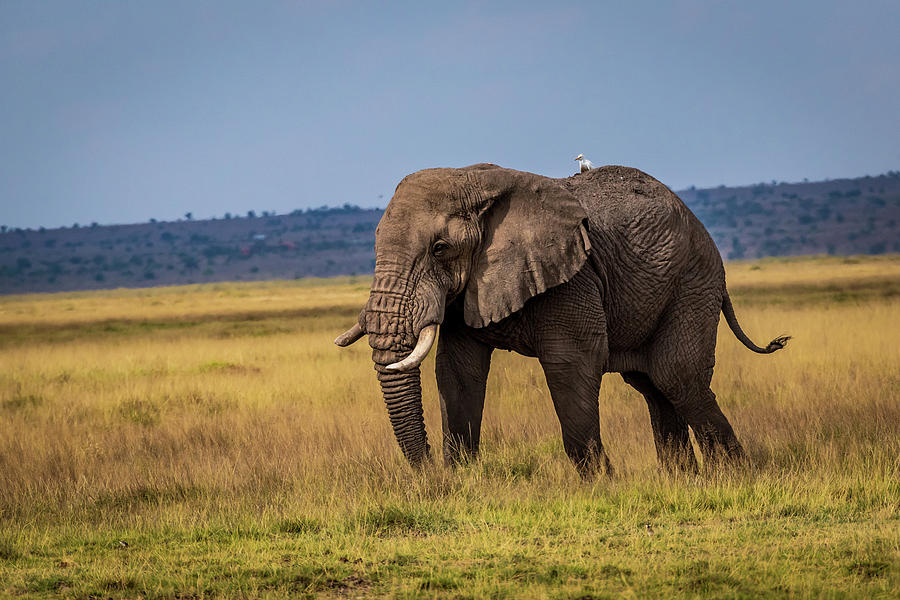The color photograph captures an African elephant in the wild, traversing the expansive savannah grassland. The elephant is depicted in a left profile stance, but its slight turn allows the right tusk to be visible, though partially broken. The animal appears either mid-stride or stationary with its trunk lowered, feeding on the greenery below. Its left tusk is clearly in view, and its tail is actively swishing, likely to ward off insects. Perched on its back is a white bird, possibly a cattle egret, known for its symbiotic relationship with elephants. The savannah, characterized by golden and greenish grasses, stretches to a low-lying hill that spans the width of the photograph. This hill, marked by dry patches and tufts of vegetation, lies under a grayish-blue sky that fills the upper part of the image, lending a serene backdrop to the scene. The elephant stands alone in the frame, emphasizing its solitary presence in this vast and open landscape.